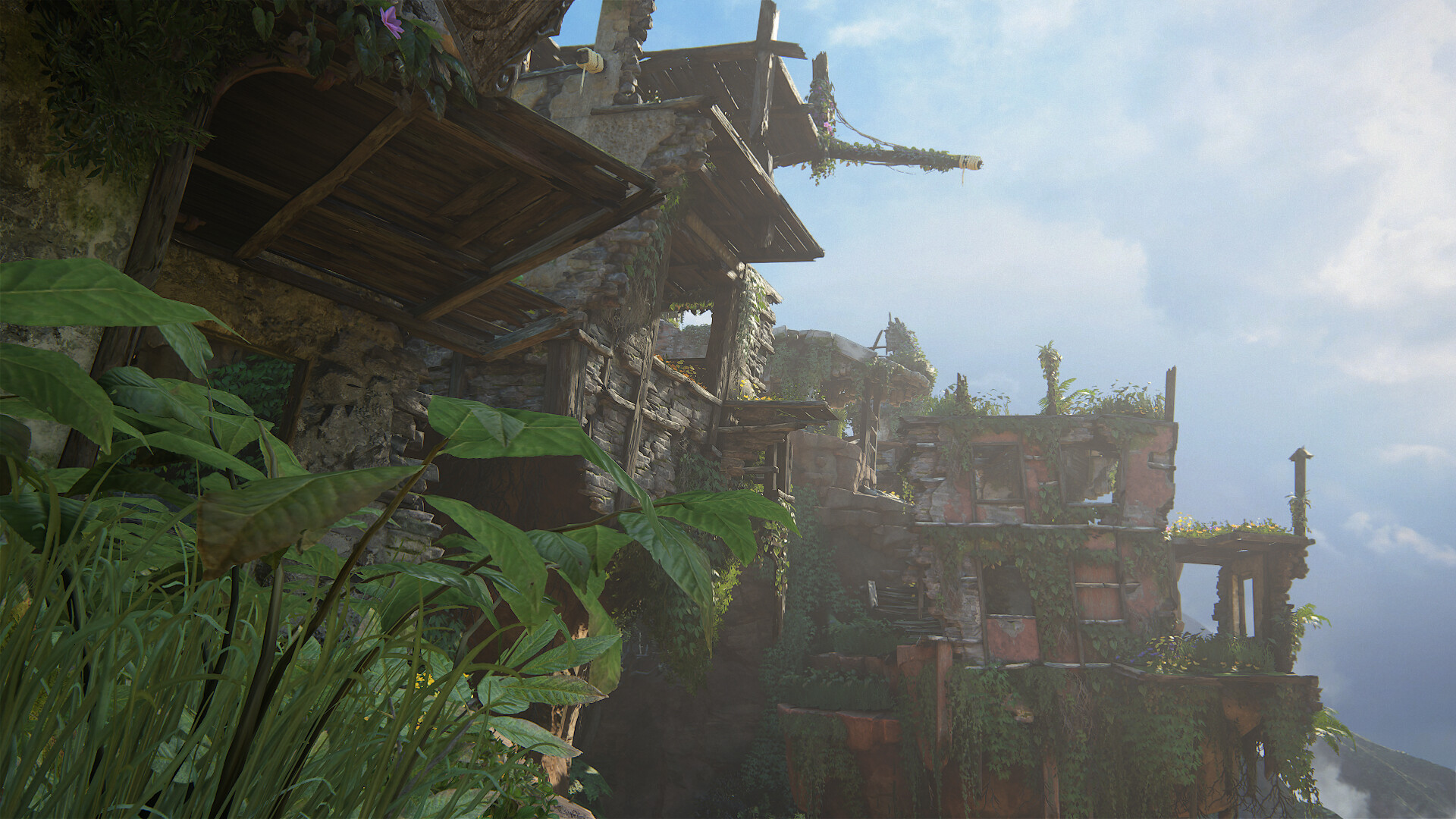This detailed screenshot from a video game, likely Uncharted 2 or 3, showcases a dramatic, dilapidated structure built into a cliffside. The scene captures a large, half-constructed or abandoned ruin with various platforms that protagonist Nathan Drake could potentially jump on and climb. The entire area is heavily overgrown with lush greenery, including moss, grass, and leaves that have enveloped the decaying wooden platforms and stone sections of the ruins. The sky occupies a significant portion of the image, stretching from the top middle to the bottom right, displaying a gradient of blue interspersed with fluffy white clouds that darken slightly towards the bottom. To the right, a distinct pinkish building stands out with detailed pots or segmented parts, contributing to the texture of the ruins. The vegetation is pervasive throughout, highlighted by clusters of green plants, some adorned with tiny white and yellow flowers. The scene exudes a feeling of abandonment and nature reclaiming its space, as the remnants of what once might have been a vibrant habitation now crumble amidst the verdant backdrop.